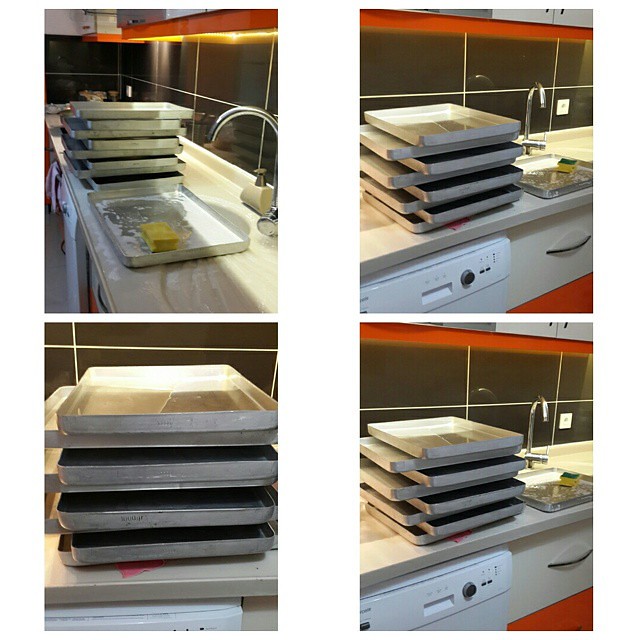The image is a grid of four photographs taken from different angles of a kitchen counter with four metal baking trays stacked in alternating orientations like linking logs. The photos do not align in the center, creating a large white negative space. The countertop is white with a black tile backsplash featuring white grout. Beneath the counter, a portion of a white appliance and drawers are visible, including red cabinets and orange trim on the upper cabinets, with light shining down from beneath them onto the sink area. One of the trays is being cleaned with a yellow sponge with a green scrubber, still covered in sudsy water. An arched faucet is also visible over the sink, indicating someone is in the process of washing and drying the baking trays.